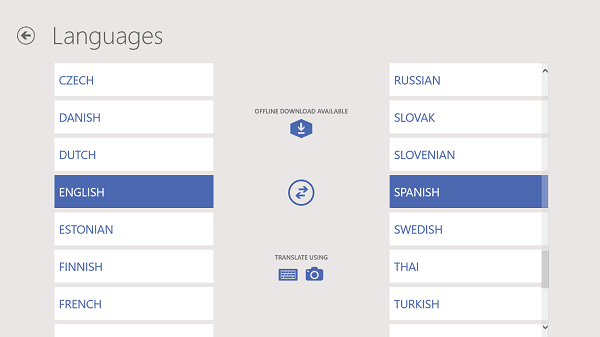The image is a screenshot, likely from a website or an app, showcasing a settings page dedicated to language options. The background is a light grey with a rectangular format. At the top left, the word "Languages" appears in a large, darker grey font, accompanied by a left-pointing arrow.

The settings page is organized into two columns of white boxes, each containing the name of a different language. The left column lists Czech, Danish, Dutch, English, Estonian, Finnish, and French. The right column lists Russian, Slovak, Slovenian, Spanish, Swedish, Thai, and Turkish. Each language is presented in blue font except for the selected ones, which are highlighted with a blue background and white text. In this instance, English is selected in the left column, and Spanish is selected in the right column.

Centered between the two columns, there's a section labeled "Offline download available" with additional text indicating "translate user." This section also includes icons for a keyboard and a camera, and horizontal arrows pointing left and right, suggesting navigational functionality. The overall layout is clean and functional, designed to facilitate easy selection of languages and additional settings-based actions.